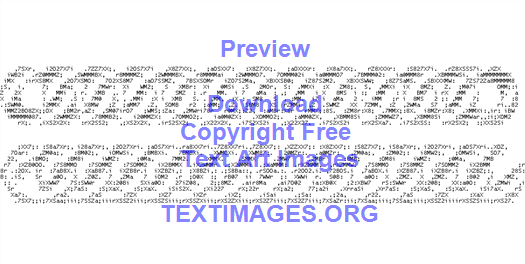This image features a promotional graphic with a white background, centered around an intricate text art illustration. At the heart of the image are two parallel, chain-like forms that stretch horizontally across the center. These forms resemble twisted dough or elongated subway bread, created entirely from densely packed keyboard characters in black ink. The tops of these forms have divots, lending a spiral, twisted appearance. Overlaying this text art is a series of blue text labels: "preview" at the top, then "download," "copyright-free," and "text art images" spaced sequentially downwards. At the bottom, the URL "textimages.org" is displayed. The placement of each text line is meticulously designed to overlap or fit within the spaces of the text art, maintaining a clean and organized look. A watermark also marks the background, repeating the URL "preview download copyright-free text art images textimages.org" faintly, ensuring the source of the creation is consistently branded.